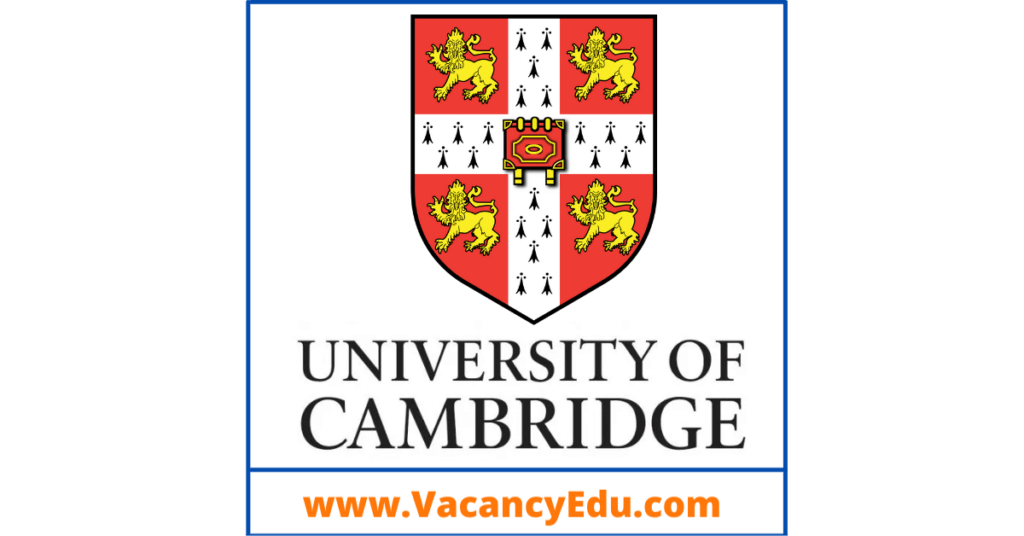This image features the emblem of the University of Cambridge, prominently displayed against a white background. The emblem is encapsulated within a thin blue border, and at the top, it prominently features the University's coat of arms. The shield displays four yellow lions situated in each corner against a reddish-orange background. A white cross divides the shield, and additional black decorations are intricately designed within the central red areas of the shield, which has a black border. 

Beneath the shield, in large, bold black letters, are the words "UNIVERSITY OF CAMBRIDGE," centered for emphasis. Below these words is a thin horizontal blue line, which forms a small box. Within this box, in orange text, is the website link "www.vacancyedu.com," adding a modern touch to the historic insignia. The overall layout, held together by clean lines and consistent coloring, reflects the prestigious and storied tradition of the University of Cambridge with a modern informational twist.